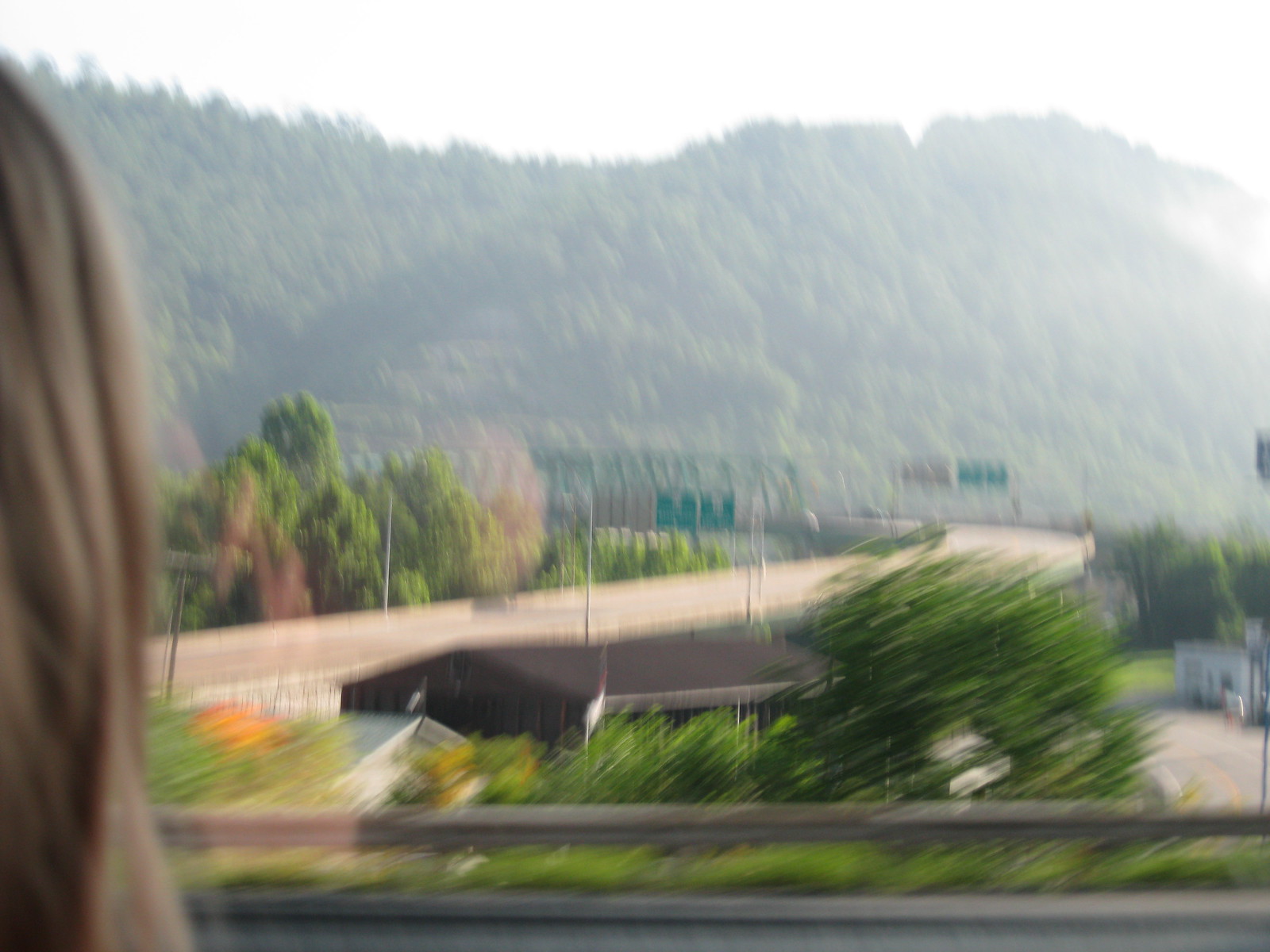The photograph appears to have been taken while in motion, resulting in a notably blurry image. The scene is dominated by lush greenery, with a large mountain densely covered in trees, giving it a predominantly green appearance. Central to the image is a highway, seemingly the primary focus, with visible green road signs indicating directions. The highway appears devoid of traffic as no vehicles are visible. To the side of the highway stands a sizeable black building, possibly a warehouse, although its exact purpose is unclear. The perspective suggests that the photo might have been taken from a bridge, as indicated by a glimpse of long blonde hair on the left side, possibly belonging to the photographer. Alternatively, it may have been shot from inside a vehicle, given the faint reflection of a person and the indication of a railing. The overall clarity is compromised, making definitive details hard to discern.